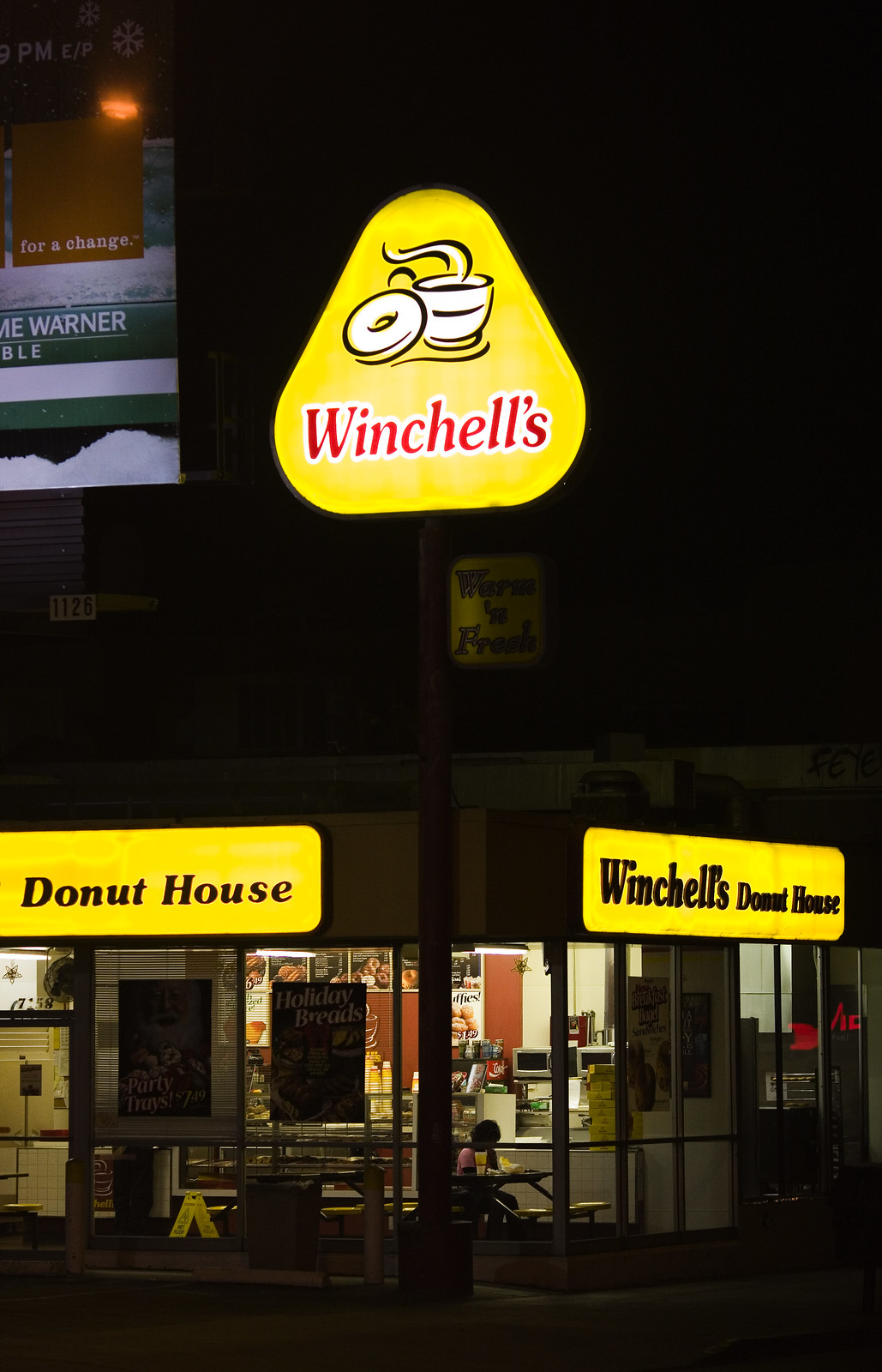The image depicts a brightly illuminated Winchell's Donut House taken from the outside at nighttime. The main focal point is the large, prominent sign atop a pole, shaped like a rounded yellow triangle with a simple illustration of a coffee cup emitting steam beside a doughnut. The name "Winchell's" is rendered in bold red letters outlined in white. The building itself is a one-story structure with large glass windows and a door to the left. The storefront features a yellow sign with "Donut House" written on the left and "Winchell's Donut House" on the right, both in black text. Through the windows, the interior is visible, showing a solitary person seated at a table, apparently with their head down, and further back, a counter area with a menu and a microwave. The image conveys a quiet, almost serene atmosphere, accentuated by the darkness of the night and the glowing lights from inside.